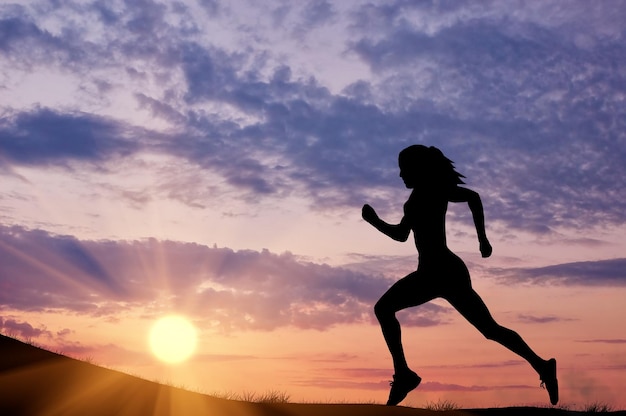The image depicts a scene at sundown, featuring a stunning photograph with a silhouetted female runner superimposed over it. The background, dominating most of the image, showcases a picturesque sunset with an open, expansive sky filled with fluffy clouds that are tinged with hues of peach, light purples, bright sunny yellows, and pale oranges. The sky transitions from a reddish bottom to a darker blue top as the sun sets, casting a serene and enchanting light over the scene. 

In the foreground, the ground appears only at the very bottom of the picture, with a few tufts of grass visible, curving slightly upwards on the lower left. Positioned prominently towards the middle and right, the black silhouette of the woman, appearing as a shadow, captures the viewer's attention. Her form is well-defined as she runs towards the left side of the image, her long hair flowing, suggesting motion and vitality against the dreamy, colorful backdrop.

The photograph is taken from a low angle, enhancing the dramatic effect of the runner's silhouette against the vibrant, setting sun and soft, cloud-filled sky, creating a captivating and dynamic visual narrative of a woman running in the twilight hours.